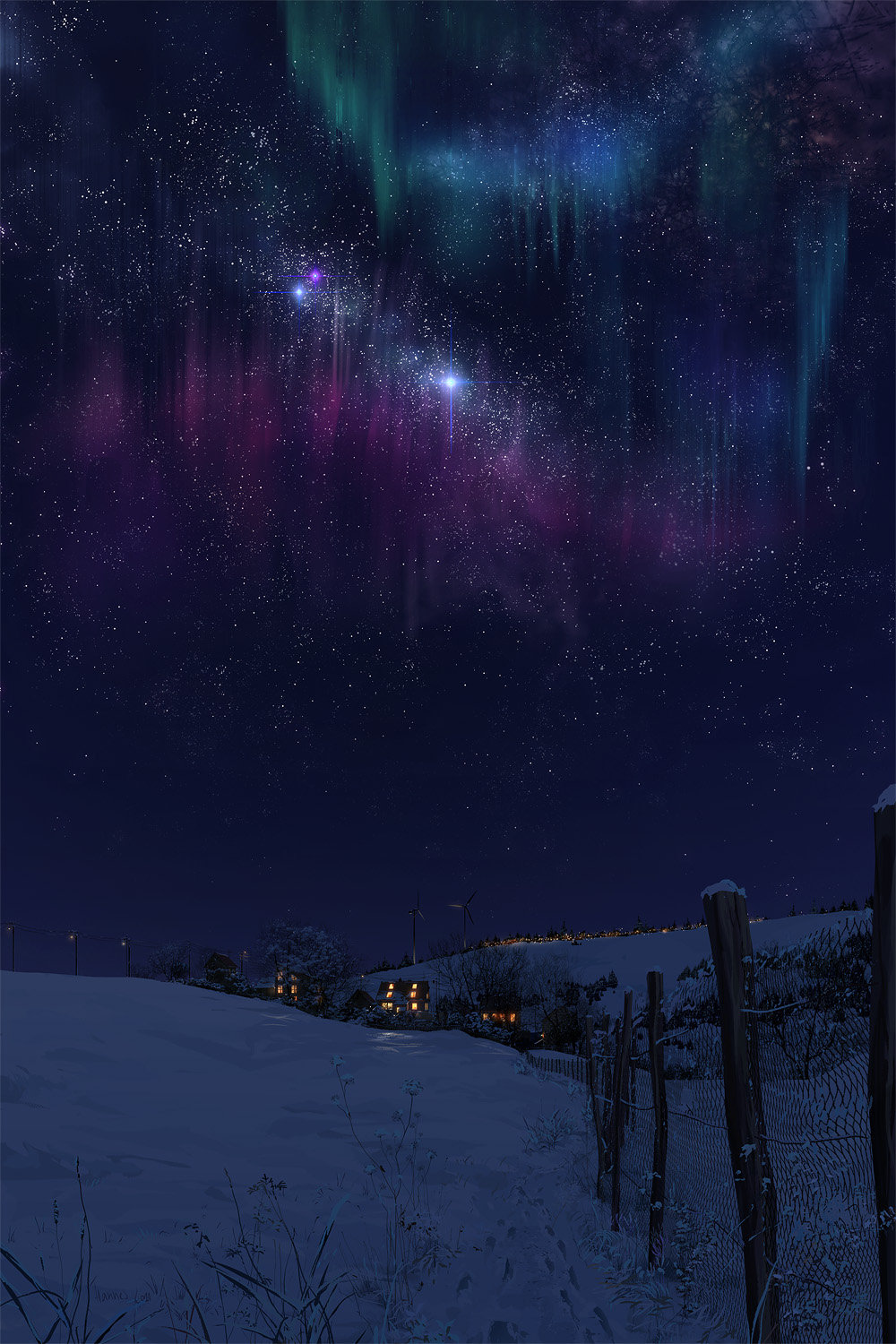A breathtaking artwork captures the ethereal beauty of the Northern Lights against a starry night sky. Set on a black canvas dotted with clusters of white stars, the scene features a mesmerizing display of the Aurora Borealis at its pinnacle. Shades of green, cascading in a U-shaped formation, blend into delicate blues, creating an otherworldly glow that extends to the northeast of the frame. Bright streaks of pink contrast vividly with the green, while a luminous white star adds to the celestial spectacle.

The Northern Lights, depicted as vibrant, undulating scribbles of pink, stretch across the horizon. Below their luminescence, a gradient of black and gray space with three twinkling stars bridges the gap between the heavens and earth. The terrestrial landscape showcases a double hill formation, with the slope of the front hill meeting an almost parallel but slightly descending rear hill. Atop these hills sit distant, quaint houses, one marked with an "ABC" sign, alongside windmills that stand as sentinels against the night.

Closer to the viewer, additional houses and a rustic wooden fence lined with chicken wire snake across the snowy ground. Each element, from the intricate play of colors in the sky to the serene, snow-covered landscape, combines to create a captivating and serene scene that celebrates the natural and whimsical beauty of the Northern Lights.